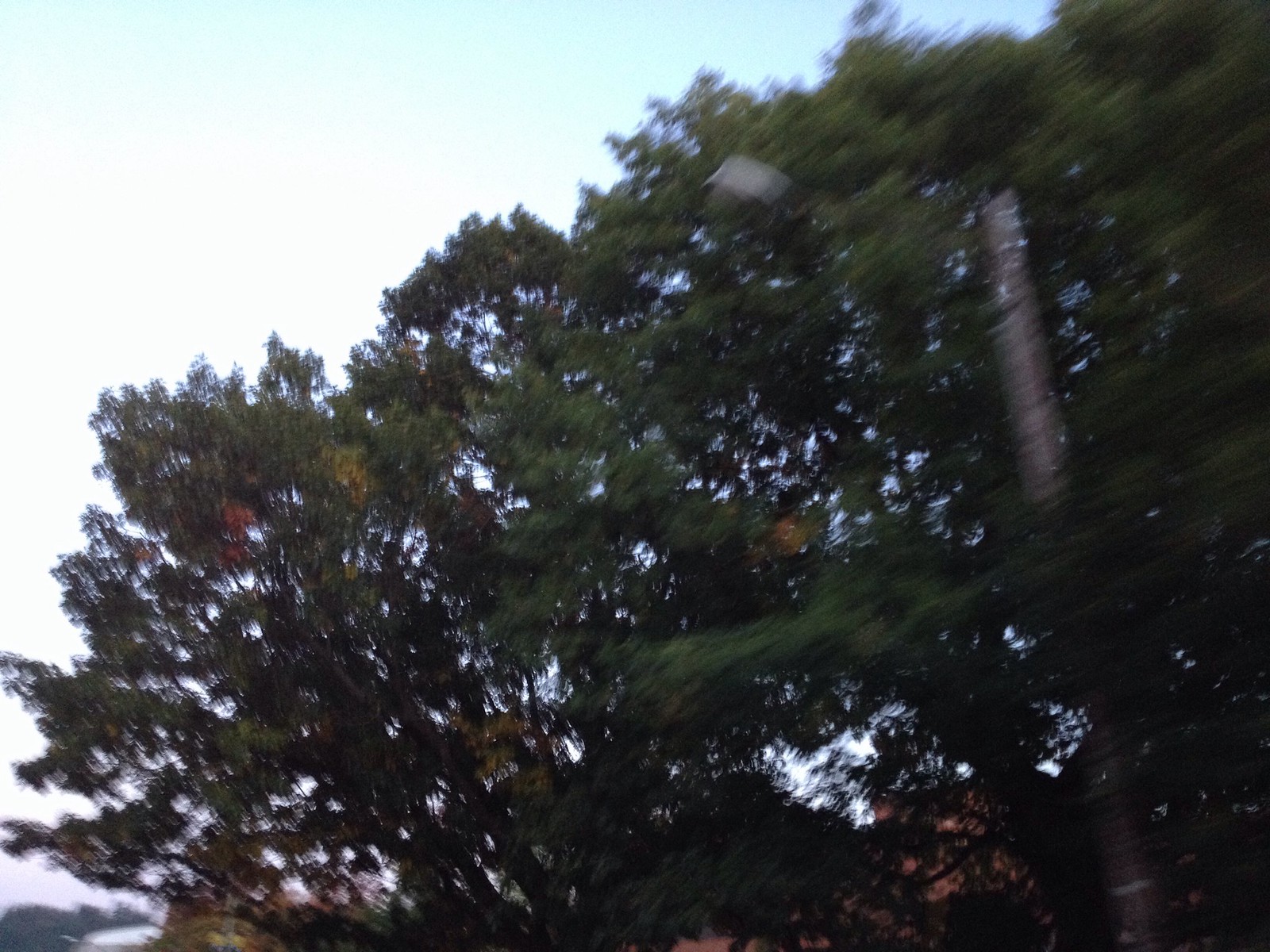The photograph captures a scene of green, leafy tree tops against a clear, bright blue sky with occasional white clouds. The image is somewhat blurry, imparting a sense of motion. Among the foliage, there appear to be multiple trees, closely grown together with leaves showing hints of orange and gold. Towards the right, partially obscured by branches, is a tall streetlight or lamppole. The light blue sky peeks through various spaces between the leaves, especially prominent in the top right corner. No people, animals, buildings, or other notable objects are present, and the photograph is notable solely for its natural, outdoor setting.